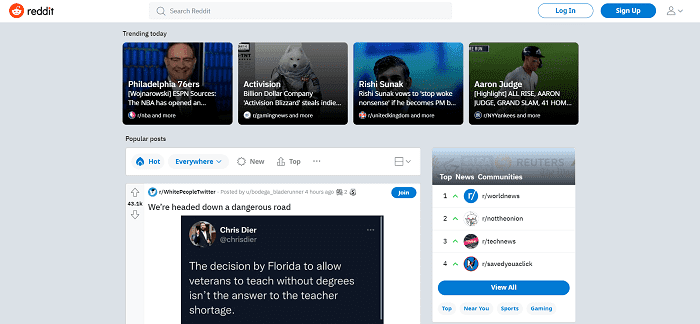This is a detailed and clean caption for the described image:

---

The image depicts a screenshot of a specific page on the Reddit website. At the very top, the white navigation bar features the Reddit logo and title at the left. Centrally located in this bar is a search field with a magnifying glass icon and the placeholder text "Search Reddit." On the far right side of the navigation bar, there are two prominent buttons: a white "Log In" button and a blue "Sign Up" button. Further to the extreme right, there's an icon representing a user profile accompanied by a dropdown arrow.

Directly below this bar, the main page begins with a section featuring four prominent cover images linked to various pages or articles. The top left corner of this section is marked by the bold text "Trending Today," indicating current popular topics or breaking news.

Beneath this section lies another bold header, "Popular Posts." Adjacent to it is a white menu bar with customizable options such as "Hot" (highlighted in blue), "New," and "Top," reflecting different sorting criteria for the posts displayed.

Scrolling further down, there is a featured post from the subreddit r/WhitePeopleTwitter. On the left side of this post, the number of upvotes, indicated by up and down arrows, reads 43.2K. Just after the subreddit title, it mentions the post was uploaded by a particular user four hours ago. The post itself is titled "We're headed down a dangerous road" and contains a screenshot of a tweet by Chris Dyer. The tweet criticizes Florida's decision to allow veterans to teach without degrees, questioning its effectiveness in addressing the teacher shortage.

Lastly, on the right side of the webpage, there is a column labeled "Top News Communities," displaying a numbered list of trending threads and a "View All" button for further exploration.

---

This caption aims to provide a comprehensive, organized, and detailed description of the image.